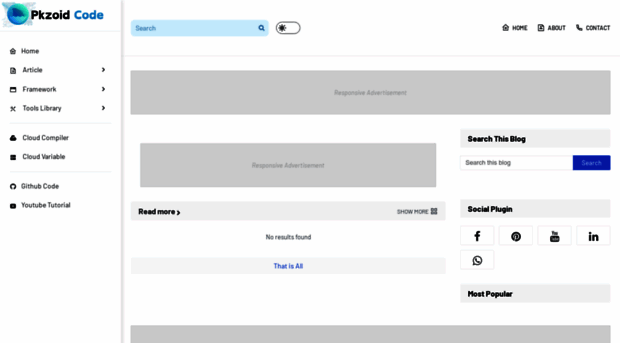This desktop screenshot captures a platform interface, likely for web development or content management, without revealing the browser, web address, or operating system. On the top left, a pale bluish-green circle featuring a small, unclear icon—possibly a Wi-Fi symbol—accompanies the label "PKZOID code." Below it, various navigation options are displayed vertically, each with an accompanying icon and an arrow signaling more choices:

- **Home**: Represented by a house icon.
- **Article**: Denoted by a piece of paper.
- **Framework**: Indicated by a square.
- **Tool Library**: Illustrated with a set of tools.
- **Cloud Compiler**: Marked by a cloud icon.
- **Cloud Variable**: Represented by another square-like icon.
- **GitHub Code**: Possibly indicated by a trophy-shaped icon, although the image is unclear.
- **YouTube Tutorial**: Accompanied by the recognizable YouTube logo.

On the right-hand side, an interface includes a search bar, a dark mode toggle, and navigation links for "Home," "About," and "Contact." Below these, gray frames display text that is unreadable, followed by sections labeled "Search this blog," "Read more," and "No results." The interface also features social media plugins for Facebook, Pinterest, YouTube, LinkedIn, and WhatsApp.

Overall, this screenshot seems to showcase a tool designed for creating or managing websites, offering various resources and features to support web development and content creation needs.